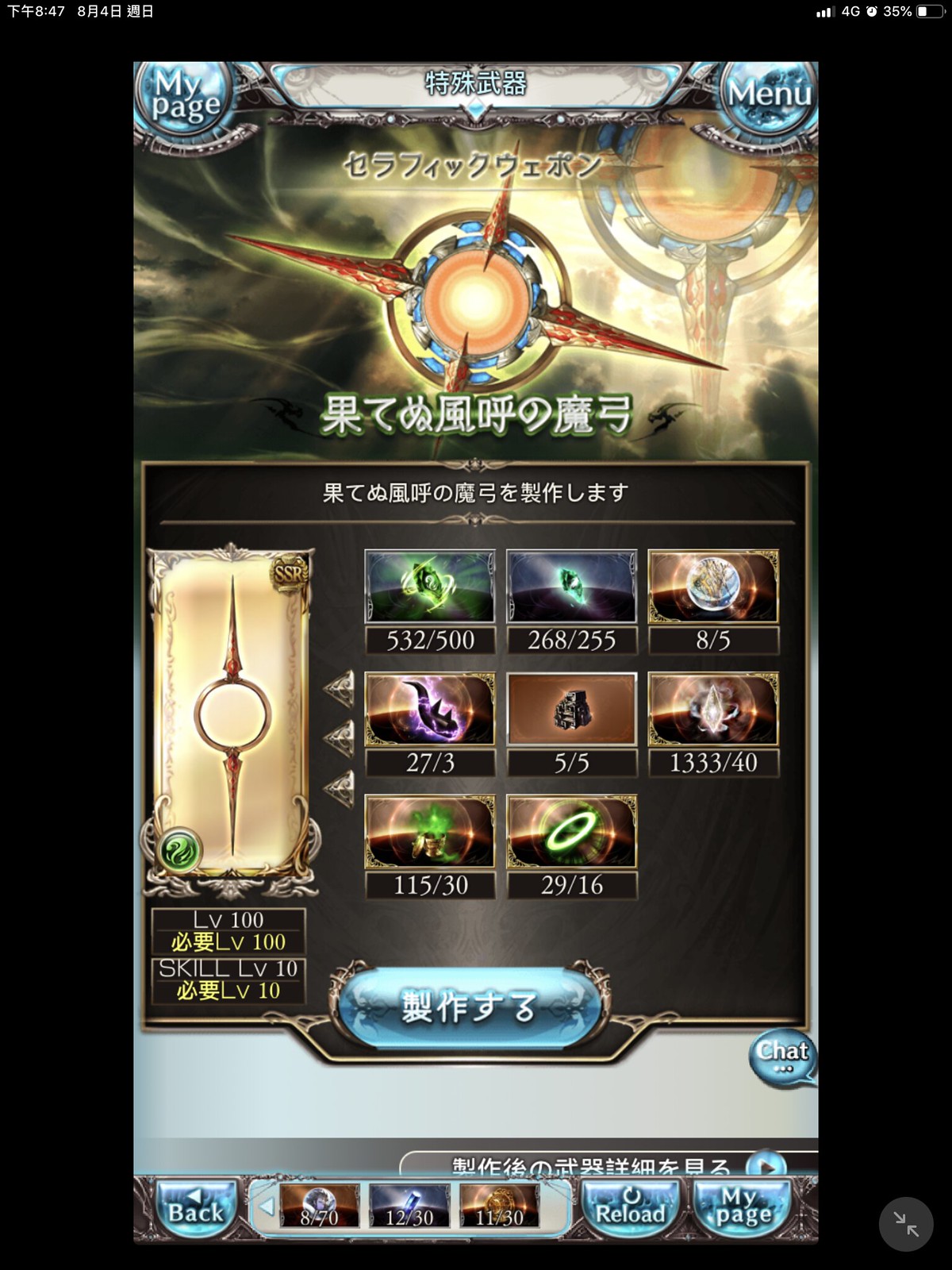The image captures a screenshot from a video game on what appears to be a tablet or phone, with a black background surrounding the screen. At the very top, there's a status bar displaying 4G service, 35% battery life, and a series of oriental symbols or Asian lettering. At the left side of this bar, there's a clock and a circular icon labeled "My Page," while the right side has a circle labeled "Menu."

Below the status bar, there is a visual that resembles a spacescape, featuring a spaceship amid blurry galaxies and clouds. Directly under this, more Asian symbols are displayed, leading into a series of eight boxes, each marked with numbers, hinting at items or skills in the game. The left side includes an icon resembling a key, indicating an important game element.

Towards the bottom, there are multiple buttons, including options labeled "My Page" and "Reload." A chat button and a circular icon with arrows pointing towards each other diagonally are also visible. The game appears to be a role-playing game (RPG) with an inventory or skill menu screen shown prominently. Here, various items, weapons, and possibly magic tools are displayed. Text indicating levels and skills are seen, with one section showing a level 100 skill level 10. To finalize selections, a blue button is available, reinforcing the RPG mechanics of leveling up and managing items.